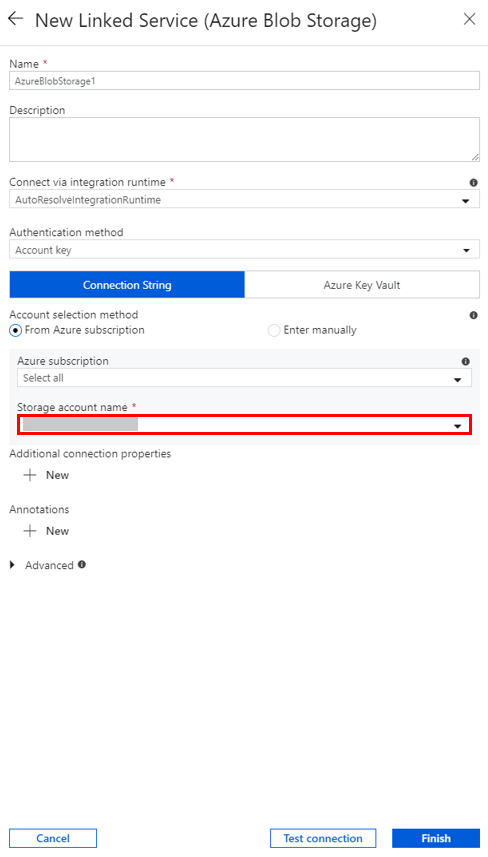The screenshot depicts a detailed form for creating a "New Linked Service" with Azure Blob Storage in a data management application. 

In the upper left-hand corner, there is a back arrow with the label "New Linked Service (Azure Blob Storage)" beside it. The upper right-hand corner features a close button (X). 

The form begins with a field labeled "Name," filled in with "Azure Blob Storage 1." The following field is "Description," which includes a resizable text area marked by an expandable corner indicator located at the bottom right.

Continuing down, the next row is "Connect via Integration Runtime," marked with a red asterisk and accompanied by an information icon (i) at the end. The text "Auto Resolve Integration Runtime" is filled in, alongside a dropdown arrow for selection.

Further down, "Authentication Method" shows "Account Key" as the chosen method, with an associated dropdown arrow for other options. Below this, there are two buttons side-by-side: the left button, which is blue with small lettering saying "Connection String," and another on the right reading "Azure Key Vault" in smaller text, both buttons seemingly surrounded by unnecessary blue space.

The form then presents an "Account Selection Method" with a toggle button featuring two options: "From Azure Subscription," which is the selected option marked by a black circle with a blue outline, and "Enter Manually," which is not selected. 

Beneath this toggle, there is a gray background section labeled "Azure Subscription," with "Select All" chosen, indicated by a downward arrow.

A key part of the form is highlighted in red to indicate its importance. This section, labeled "Storage Account Name" with a red asterisk, is partially obscured by a gray mark but includes a dropdown menu.

The last sections in the form include areas for "Additional Annotations" and "Advanced" options.

Finally, the form concludes with three buttons: "Cancel," "Test Connection," and a blue "Finish" button at the bottom.